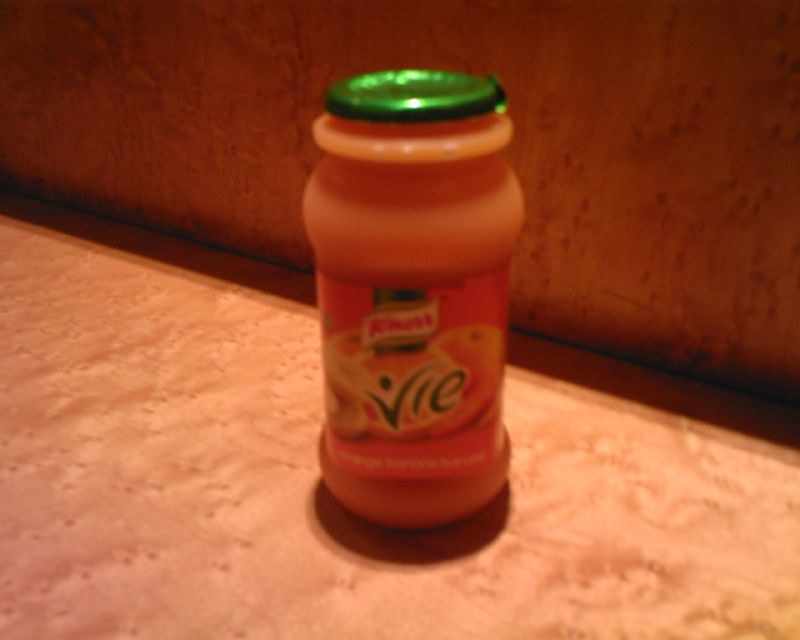The image depicts a somewhat blurry, close-up of a drink bottle that appears to be a fruit beverage. The bottle is peach-colored, possibly due to the liquid within, but the color hints at a darker, brownish-orange hue, potentially resembling carrot juice. The label prominently displays the text "VIE" with a dot above the "V," evoking imagery of a person's head with arms raised. Above this text is the green Knorr logo, though it is not entirely clear. The bottle has a bulbous shape with a gold foil cap that appears vacuum sealed. Additionally, the label features some fruits, including oranges, which may contribute to the darkened tone of the liquid. The bottle rests on a textured, light-brown surface, akin to knotted wood, and is situated in front of what looks like a rust-colored upholstered backrest, similar to a park bench or booth cushion, adding to the cozy ambiance of the scene.